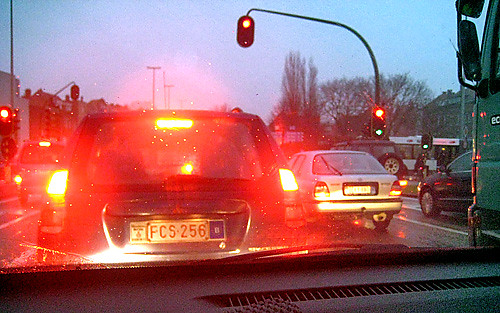Taken from inside a car, this photo captures an urban scene at a busy intersection. The top of the dashboard and a portion of the windshield frame the view. Directly ahead, a small blue car, bearing the license plate FCS256, waits at a stoplight. To the right of the blue car, a large green truck begins to come into view, followed by a silver or white car, a black sedan, and a Jeep further ahead. 

The right turn lane is signaled by a green arrow, while the main stoplight remains red. In the background on the right-hand side, a cluster of trees and a single building can be seen. The left-hand side features a series of buildings stretching down the street, adding depth to the urban landscape.